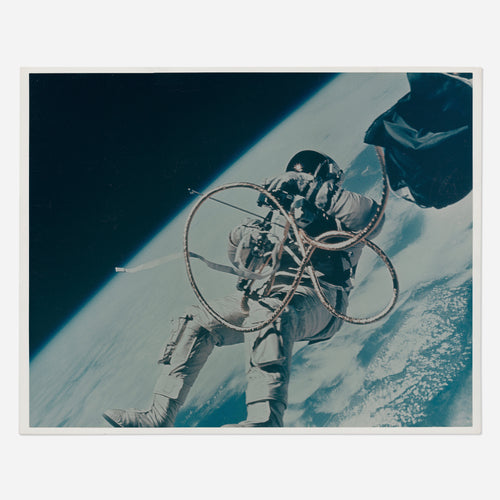The image depicts an astronaut in a white spacesuit, with their sun visor down, engaged in a spacewalk. The astronaut is floating in the dark expanse of space, with the blackness of the universe occupying the upper left corner of the frame. Below him, the Earth is visible, showcasing the blue of the ocean, the curvature of the planet, and scattered clouds.

There are several tubes and straps connected to the astronaut. A prominent silvery tube extends from the astronaut to the upper right of the image, likely linked to part of the space shuttle, some of which is partially visible, albeit only a small segment. One strap appears loose, trailing to the side, while another, less distinctly identified, seems to pull away from him. 

The overall composition suggests the astronaut might be performing repairs on the space shuttle, surrounded by the awe-inspiring, juxtaposing visuals of the vibrant Earth below and the deep, starless black of space above. The photograph offers a captivating snapshot of human endeavor against the backdrop of the vast cosmos. The image appears like it could belong to a photo album or a framed photograph, emphasizing its significance.